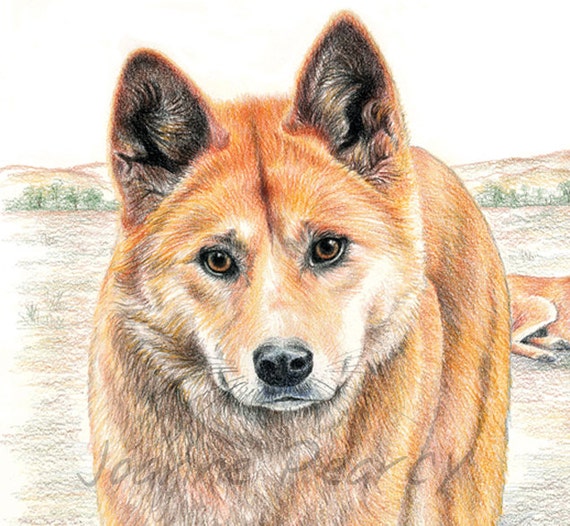This detailed drawing by Joanne Percy depicts a red fox with strikingly bright eyes and long ears, prominently gazing at the viewer. The red fox, meticulously drawn, exudes a sense of joy and contentment, with its whiskers and a delicate smile adding to its lively expression. The background features lush greenery with trees, bushes, and rolling plains, where another animal, likely another fox, is partially visible. This second animal's hind legs and paws can be seen, blending harmoniously with the natural setting. The focus remains on the central fox, thoughtfully illustrated with attention to detail, making it a mesmerizing piece.